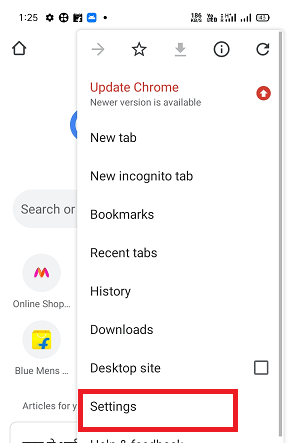The image is a cell phone screenshot displaying a web browser interface, specifically Google Chrome. 

In the upper left-hand corner, the time is displayed as "1:25" in gray. Adjacent to the time from left to right are: 
- A black settings icon,
- A gray circle with white dots (possibly a notification or menu icon), 
- A gray rectangular placeholder, 
- And a blue box featuring a white icon in its center.

On the right side of the status bar, in gray, are indicators for battery life, reception, and Wi-Fi status.

The main content of the screen shows an open browser window occupying about two-thirds of the screen on the right. There is white space on the left side. The browser window is outlined in light gray and features a row of icons at the top:
- A right-pointing gray arrow,
- A star (likely for bookmarks),
- A download icon (arrow with a line),
- A black circle with an eye in the center (possibly a privacy or incognito mode indicator),
- And a reload icon (almost complete circle with an arrow).

Approximately three lines down from the top, bold red text commands attention with the phrase "Update Chrome." Below that, black text reads, "A newer version is available." To the right, a red circle with a white upward-pointing arrow suggests an actionable update.

Further down is a list in gray text, which includes options such as:
- New Tab,
- New Incognito Tab,
- Bookmarks,
- Recent Tabs,
- History,
- Downloads, 
- Desktop Site,
- Settings.

Notably, "Settings" is highlighted with a thick red rectangle drawn around it.

In the left section of the screen just where "New Tab" begins, a blue half-circle is visible. The center of the screen displays part of a gray oval with the word "Search" inside it.

At the bottom of the screenshot are two visible icons labeled "Offline Shop" and "Blue Men's," hinting at shortcuts to specific apps or services.